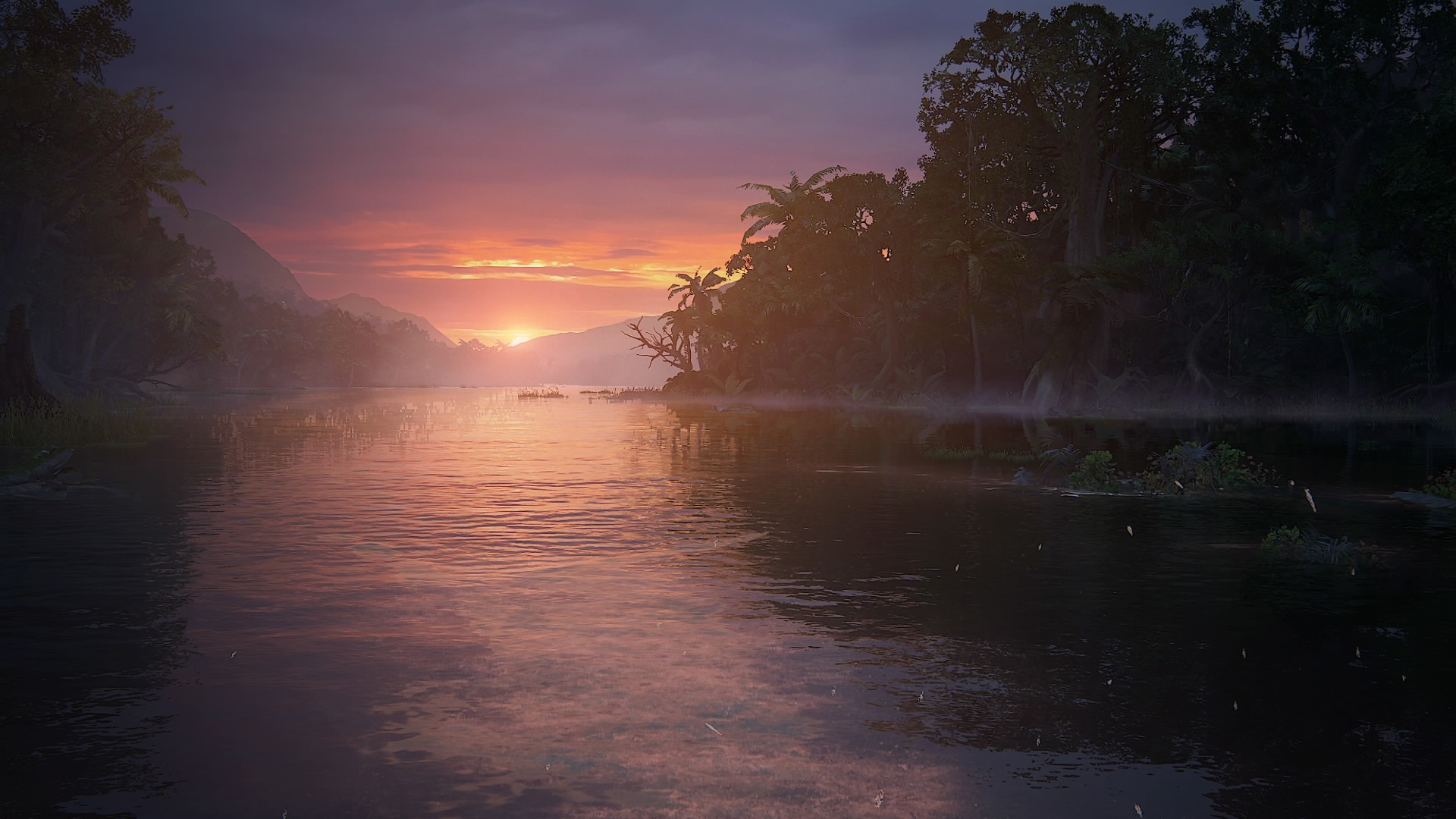This exquisitely captured image, potentially a product of professional photography or AI generation, showcases a breathtaking tropical scene. The focal point is a serene river, with the vantage point taken from its center, offering an immersive view. Majestic tropical trees frame both sides of the riverbank, their forms silhouetted against the vividly colored sky, which glows with hues of purple, pink, and orange, suggesting either a sunrise or a sunset. The shallow waters of the riverbed are dotted with reeds, adding texture to the tranquil surface. In the distance, a few clouds pepper the horizon near some gentle, looming mountains, which contribute to the scene's depth and grandeur. This lush, vibrant landscape exudes natural beauty and tranquility, making it a captivating and picturesque setting.